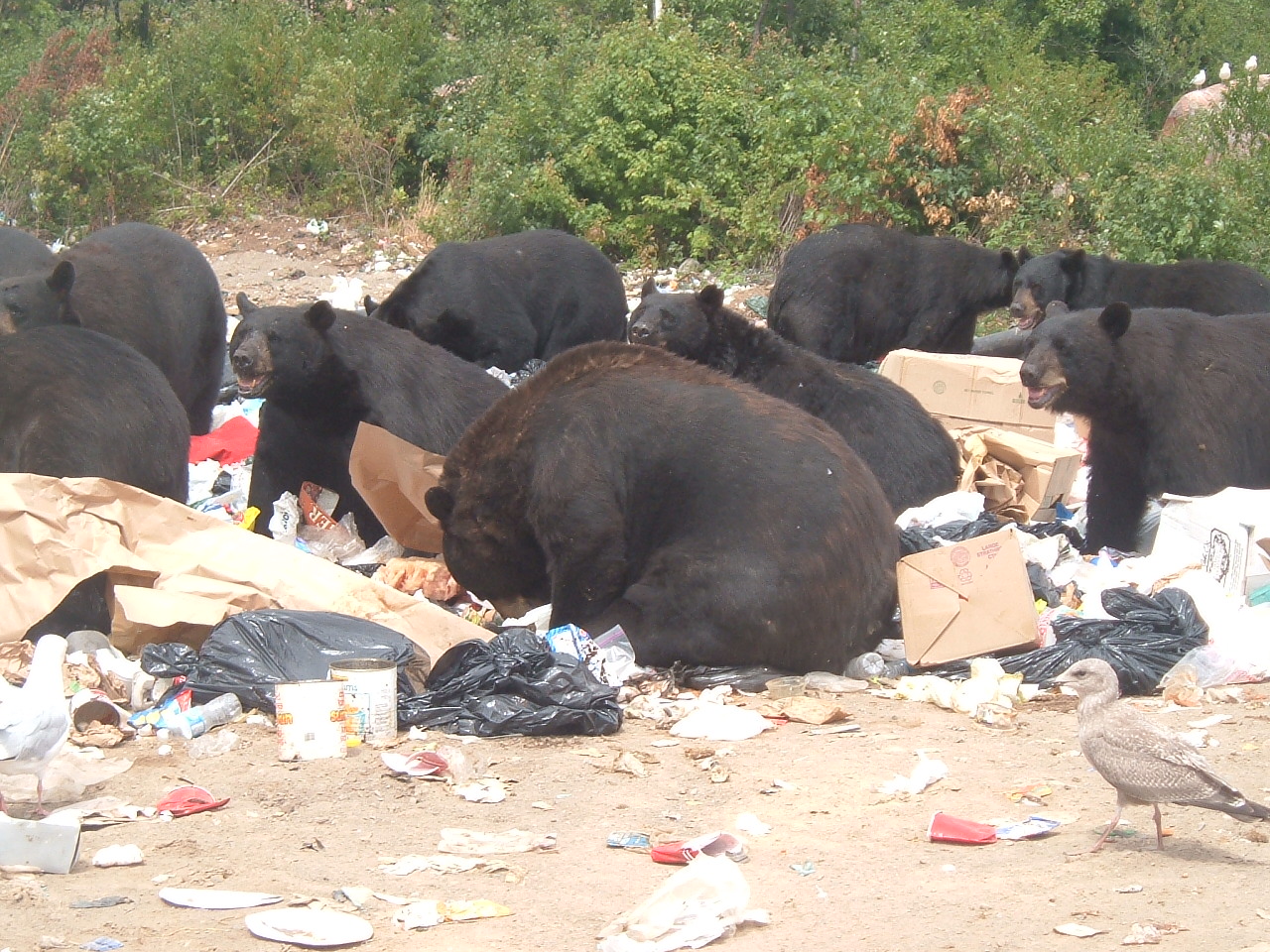The photograph captures a chaotic scene at what appears to be a landfill or dumping site, strewn with various types of refuse, including water cups, drink cans, crumpled packaging, paint cans, and trash bags. Amidst this sea of garbage, nine large black bears forage for food. Some bears are standing while others are sitting or have their heads down, intently searching through the litter. The terrain they occupy is sandy, adding to the disarray. In the lower right corner of the image, a seagull walks from right to left, and another seagull is visible on the bottom left edge of the frame. The background is characterized by green vegetation, including bushes and low hedges, with a few other birds dotting the scene, completing this vivid portrayal of wildlife interacting with human waste.